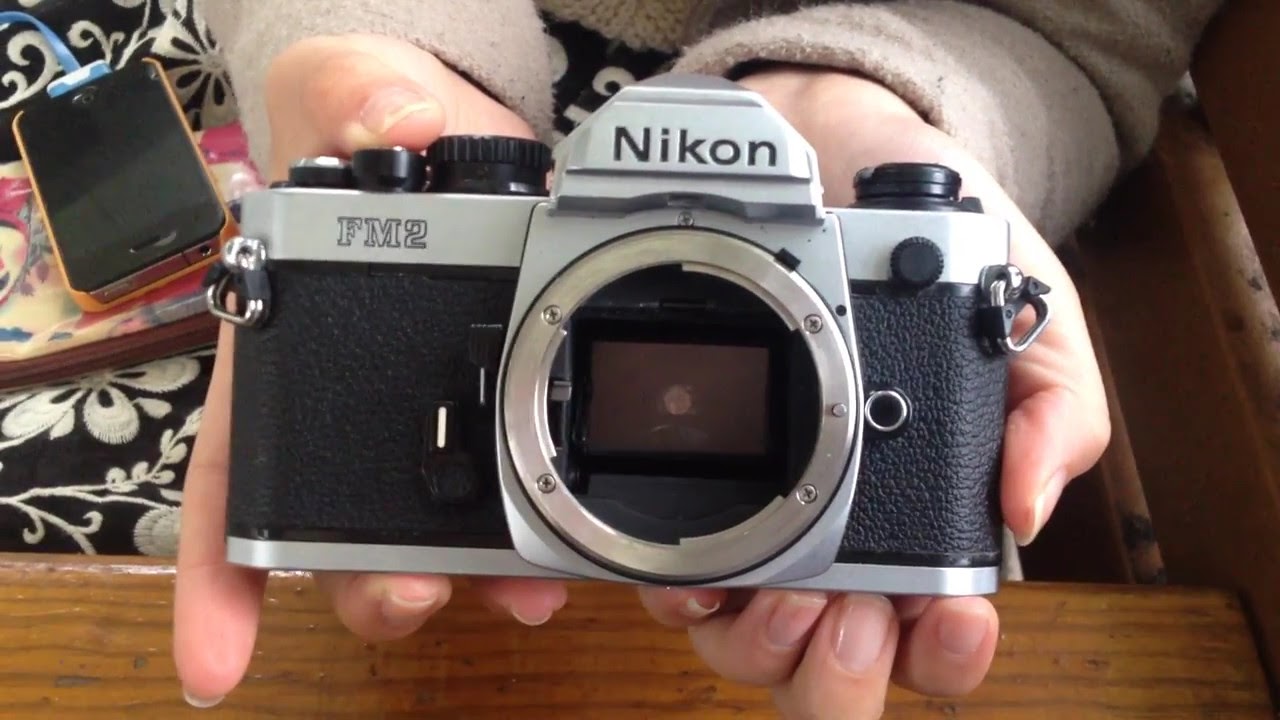In this detailed indoor photograph, a pair of hands holding a Nikon FM2 single-lens reflex camera is the focal point. The camera, which features a black body with silver borders and the word "Nikon" inscribed on it, is held by hands emerging from the sleeves of a light brown, long-sleeve shirt. The individual, who appears to be either Asian or white, is not visible beyond their hands. To the left of the camera lies a smartphone in a pink or orange case, attached to a charging cable. The person is seated on a piece of furniture, possibly a sofa or chair, adorned with a black upholstery that features white floral patterns. A wooden object is partially visible at the bottom and to the side of the image, adding more context to the setting.